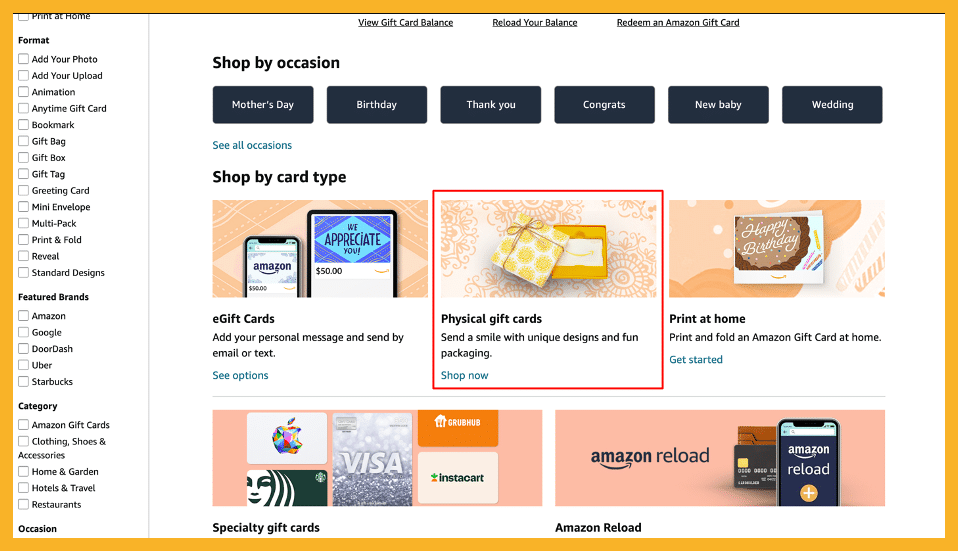The screenshot captures a webpage with an orange border framing the entire image. On the left-hand side, a vertical menu lists several categories and options, including:
- Print at Home
- Format
- Add Your Photo
- Add Your Upload
- Animation
- Anytime Gift Card
- Bookmark
- Gift Bag
- Gift Box
- Gift Tag
- Greeting Card
- Mini Envelope
- Multi-Pack
- Print and Fold
- Reveal
- Standard Designs
- Featured Brands (such as Amazon, Google, DoorDash, Uber, Starbucks)
- Categories including Amazon Gift Cards, Clothing, Shoes and Accessories, Home and Garden, Hotels and Travel, Restaurants
- Occasions like Mother's Day, Birthday, Thank You, Congrats, New Baby, Wedding, See All Occasions
- Card Types including E-Gift Cards, Add Your Personal Message and Send by Email or Text, See Options

At the top right, additional options are displayed:
- View Gift Card Balance
- Reload Your Balance
- Redeem an Amazon Gift Card
- Shop by Occasion 

The image includes varied visual elements, prominently featuring electronic devices displaying Amazon gift cards. On the left, a smartphone showcases an Amazon Gift Card with a value of $50. Adjacent to it, a tablet features another Amazon Gift Card adorned with the message "We Appreciate You" for $50.

In the center, a physical gift card is presented inside an elegant gift box. The box lid has a white background decorated with yellow polka dots and is tied with an ornamental gold bow positioned at the top left corner. This boxed card is set on a patterned surface, accompanied by a caption saying, "Physical Gift Card, Send a Smile with Unique Designs and Fun Packaging, Shop Now," highlighted by a red outline.

Additionally, an image of a gift card with a chocolate cake design is incorporated, displaying the text "Happy Birthday" in white, with multicolored sprinkles and birthday candles at the bottom right of the cake. It invites users to "Print at Home, Print and Fold an Amazon Gift Card at Home, Get Started."

At the bottom of the screenshot, images of various specialty gift cards (Apple, Starbucks, Visa, Grubhub, and Instacart) are displayed alongside the label "Specialty Gift Cards."

Lastly, an "Amazon Reload" section is illustrated with a cell phone displaying the text "Amazon Reload." This phone is laid out alongside a brown leather wallet and a black credit card, further emphasizing the convenience of the "Amazon Reload" service.